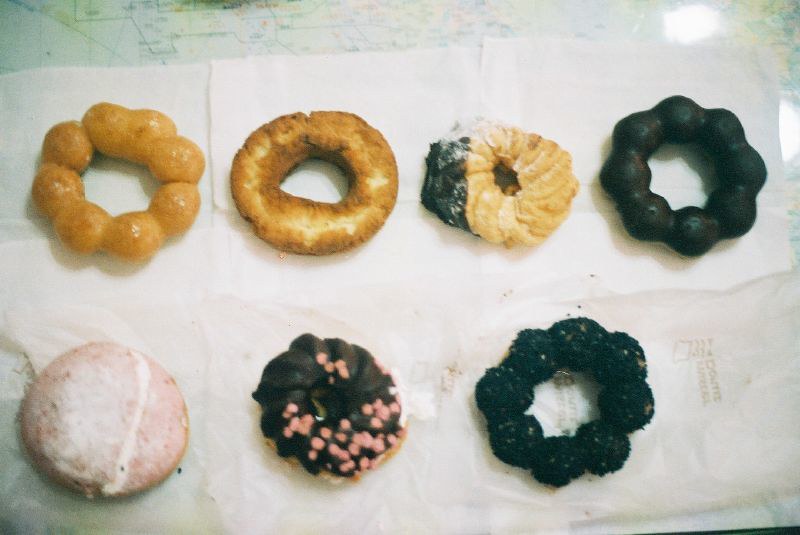The image depicts seven assorted donuts arranged on paper napkins with slight chocolate smudges, laid out on a folded road map. There are four donuts in the top row and three in the bottom row. The doughnuts themselves vary in type: starting from the top left, the first is a wreath-shaped mochi donut (pondering) with pull-apart sections. Next is a plain, un-iced donut, followed by a cruller with a dark coating, and another mochi donut but with a black glaze. The second row begins with a powdered donut, possibly strawberry-flavored, followed by a chocolate-covered cruller adorned with pink sprinkles, and ends with another mochi donut with chocolate glaze. The background features a road map, lending an out-of-focus texture, and a prominent glare in the upper right corner indicating a light source from that direction. The napkins under the donuts are white and have some text related to donuts.